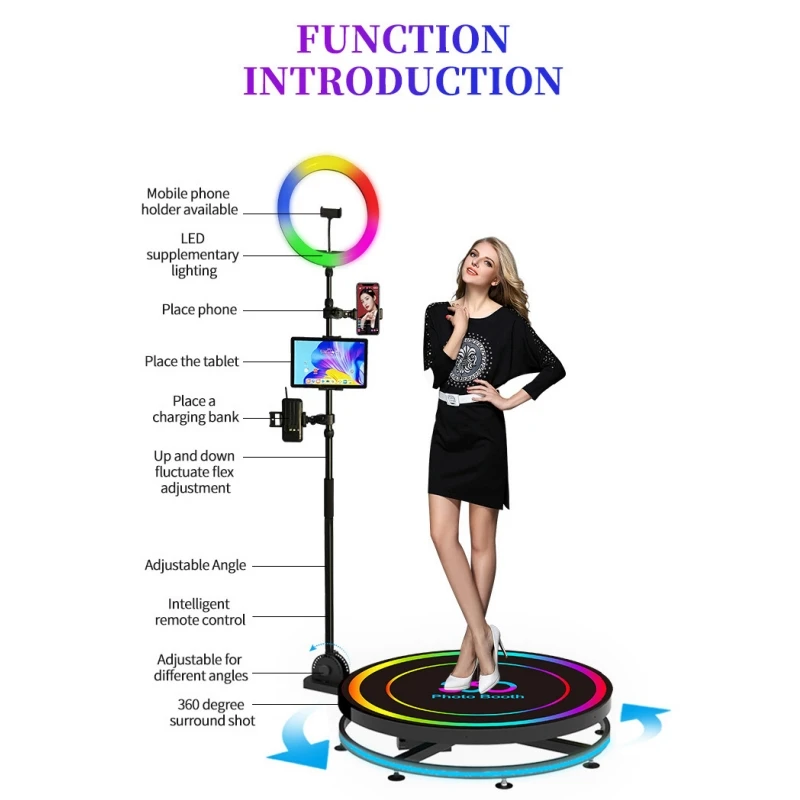The advertisement features a digital depiction of a realistic young woman with long, slightly curled blonde hair, wearing a knee-length black dress with a white belt and white heels. She's standing on a black platform with rainbow edging, highlighted by a blue ring on the pedestal base. Above her in vibrant purple and blue text, the image reads "Function Introduction." 

The stand next to her holds several devices: a mobile phone, an iPad, and a charging bank, all clearly labeled. At the top of the stand is a multicolored ring light (in shades of blue, yellow, orange, pink, green, black, and white) with the label "LED supplementary lighting." The stand is equipped with a mobile phone holder, and features various labels detailing its capabilities: "place phone," "place tablet," "place a charging bank," "up and down fluctuate flex adjustment," "adjustable angle," "intelligent remote control," and "360-degree surround shot." The background is predominantly white, making the colorful components and text stand out.